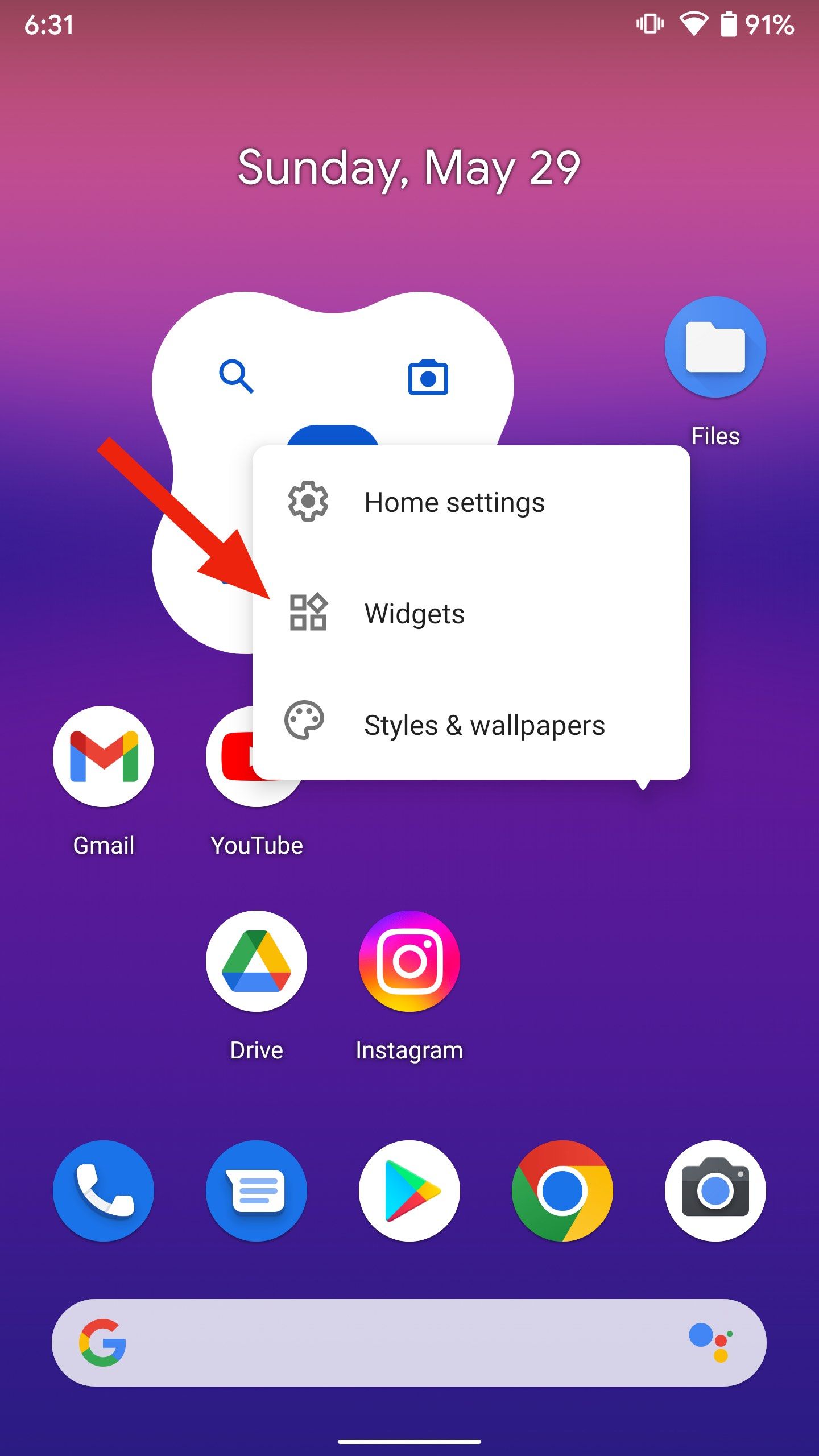This image showcases the home screen of an Android cell phone. The background features a gradient that transitions from a light purple at the top to a dark purple at the bottom. Prominently displayed in the center are the day and date in large white letters: "Sunday, May 29th." On the screen is a pop-up box, which has a white background and lists three options vertically: "Home settings," "Widgets," and "Styles and wallpapers." The "Widgets" option is highlighted by a red arrow that has been edited into the image. In the background, app icons such as Gmail, YouTube, Drive, and Instagram are visible. At the bottom of the screen, there is a horizontal row of frequently used app icons: Telephone, Messages, Google Play, Google Chrome, and Camera. Beneath these icons is a search bar with the Google logo on the left and the multicolored Google dots on the right.